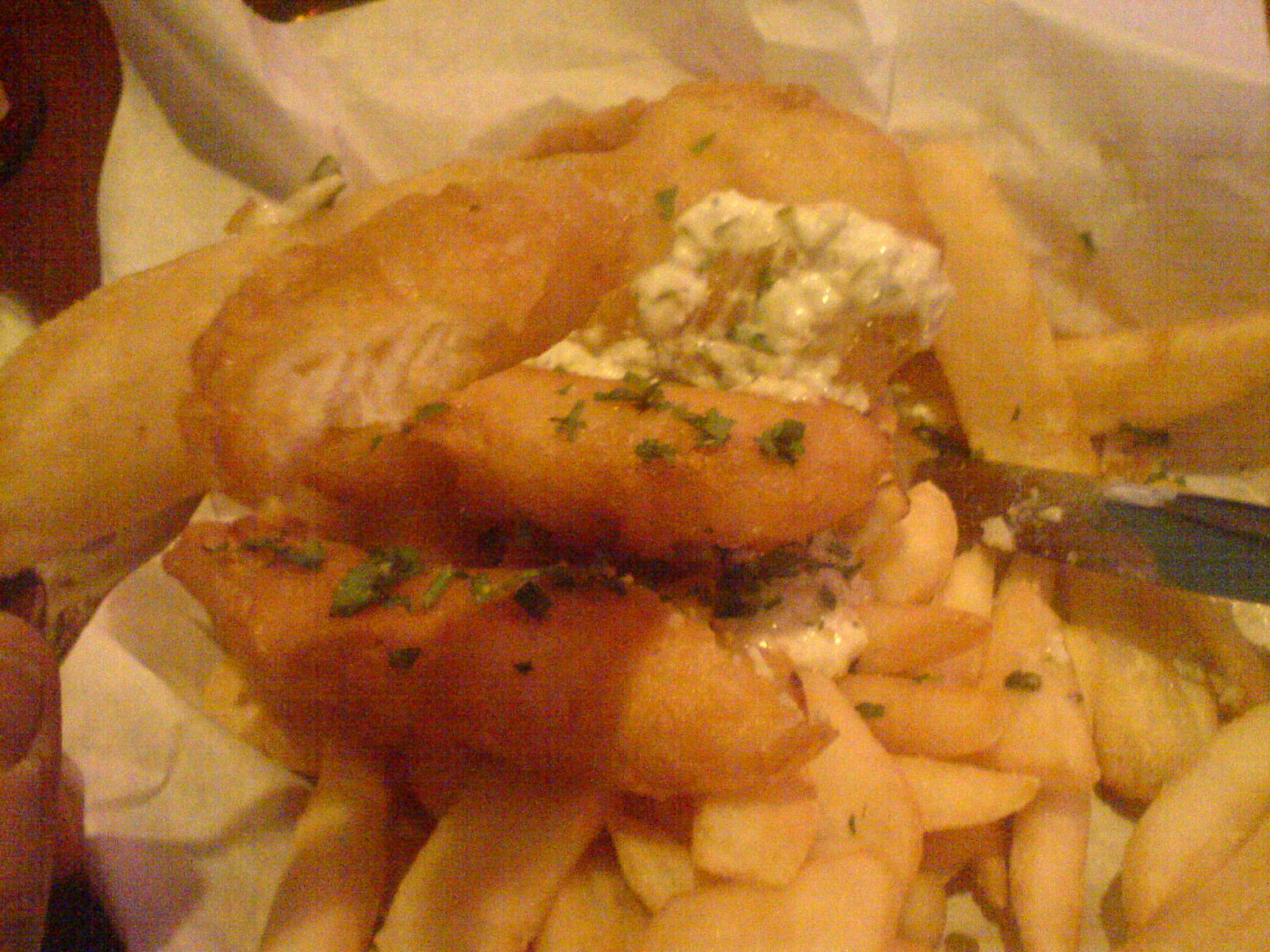The image depicts a fish and chips dinner arranged on a tray lined with white paper. A generous layer of flat-cut french fries is spread out, lightly sprinkled with green herbs and chives. Atop the fries lie three pieces of battered and fried fish, one of which has been partially bitten into or torn open, revealing its tender interior. The fish is adorned with chunky white tartar sauce, and a butter knife smeared with more tartar sauce is visible coming into frame from the right, suggesting the eater is spreading the sauce onto their meal. In the bottom left corner, a portion of the photographer's thumb and thumbnail can be seen.